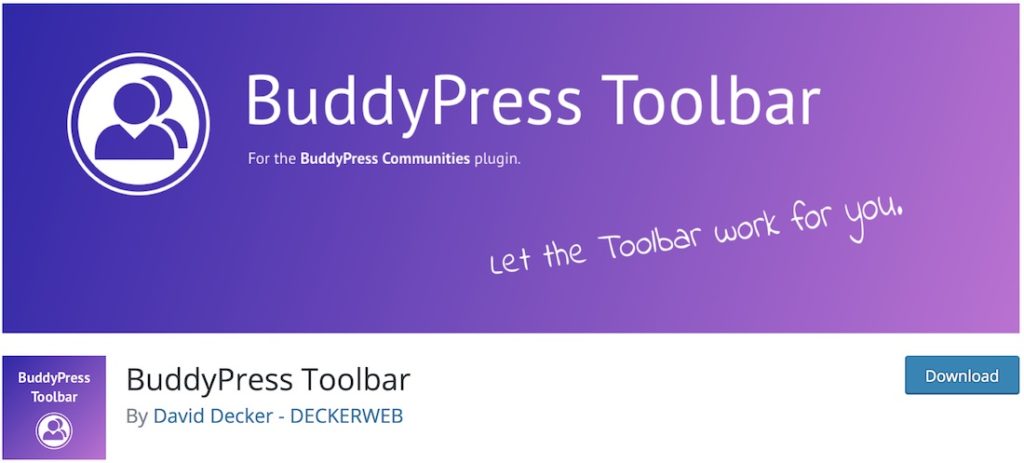The horizontal rectangular image features a striking gradient background at the top, transitioning from dark purple on the left to a light purple and finally to a purple-pink hue on the right. Prominently positioned at the top center is the text "BuddyPress" in a large, bold white font, with the letters capital "B" for Buddy and "P" for Press. Just below, a smaller, tiny white font reads "for the," followed by "BuddyPress communities" in bold white font, and "plugin" in regular white font. 

To the left of this text is the BuddyPress logo: a white circle containing two simplified human figures. Their heads are represented by purple circles, surrounded by white, and their torsos are indicated by purple shapes within the white background. The figures are encircled by a purple ring, which itself is bordered by a white ring.

Below this, on the lower half of the image, the phrase "Let the toolbar work for you" is displayed. It starts low on the left side and rises diagonally, with "for you" positioned near the middle right edge.

On the right side below the gradient area, there's a horizontal rectangular box with the word "Download" in white lettering inside. Adjacent to this, on the left side, there is a vertical rectangular box featuring a gradient from dark purple at the top to lighter purple at the bottom. "BuddyPress Toolbar" is written in white font, alongside a slightly modified version of the BuddyPress logo, this time with a pink outline instead of dark purple.

To the right of this vertical box, the text again reads "BuddyPress Toolbar" followed by "by" in a standard font, and "David Decker - DeckerWeb" in capitalized turquoise letters.